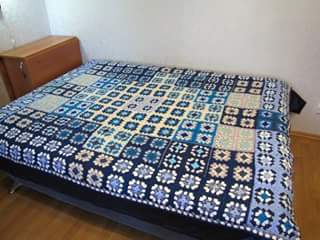This photograph depicts a cozy bedroom featuring a beautifully patterned, handmade patchwork quilt spread over a bed. The quilt is adorned with squares of varying colors, including shades of white, blue, deep blue, light green, and beige, creating a visually striking design. The deeper blue hues frame the lighter, central patterns, adding a sense of depth to the quilt. The bed, covered by this intricate piecework, is positioned against an off-white wall, noticeably absent of a headboard. Below the quilt, a deep navy bed ruffle complements the quilt's border. In the background, a small wooden cupboard, possibly concealing a radiator, adds a rustic charm to the room. The space is grounded with wood grain flooring that contrasts subtly with the room's serene palette.